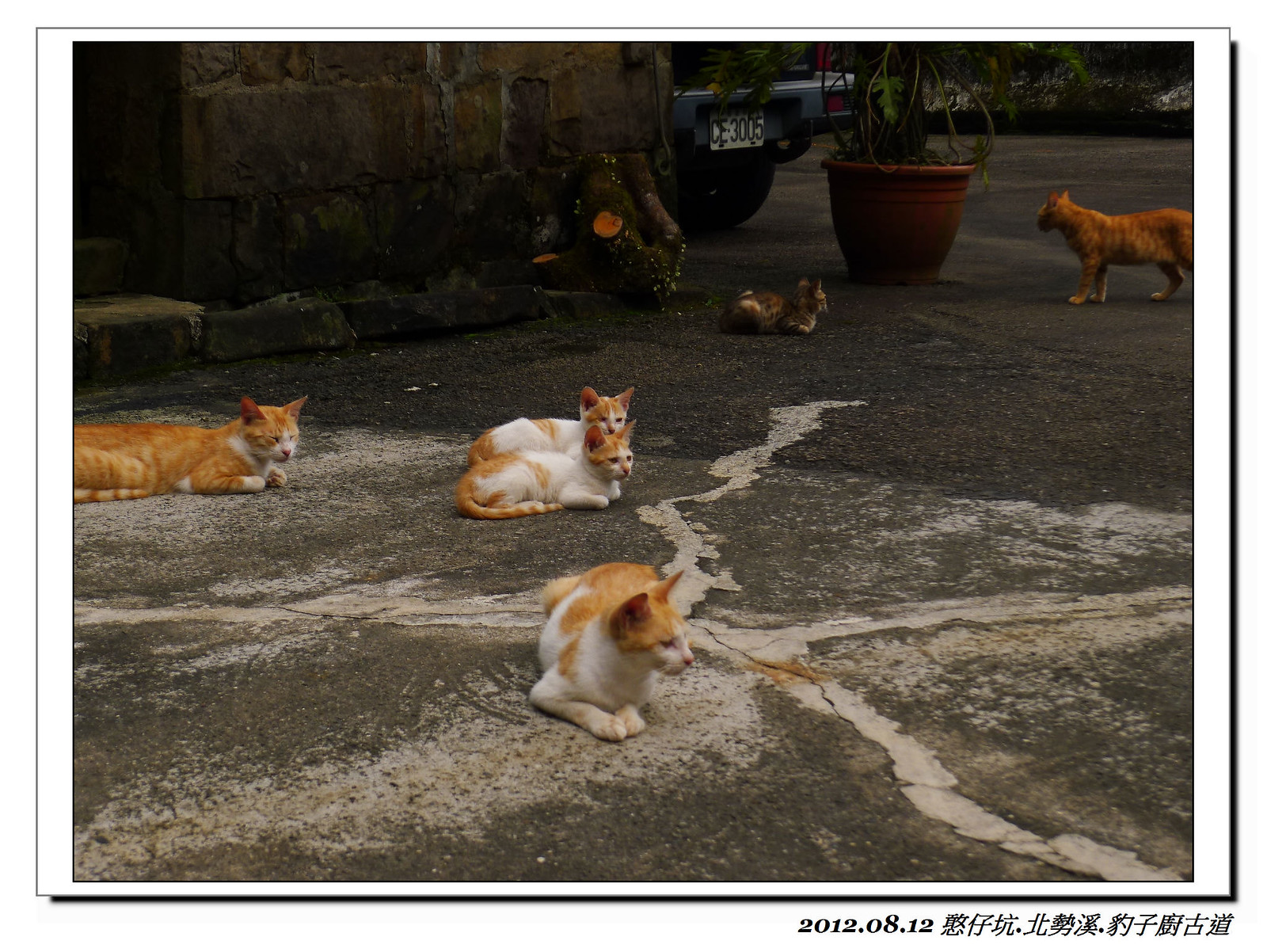The photograph, taken on 2012.08.12, showcases a tranquil outdoor scene featuring six cats in various shades of orange and white. The image captures a stone-walled building on the left side with a dark brown wooden door, and a light blue vehicle with a visible license plate reading "CE 3005." The ground is concrete with white repair marks, and a large potted palm plant sits just behind the cats.

In the foreground, four cats—mostly orange and white—are lounging peacefully, all gazing towards the right side of the picture as if something has caught their attention. One notable cat appears "loafed," with its arms tucked in and eyes closed, exuding a sense of trust and safety. Behind them, another cat is positioned near the plant pot, standing on its paws, entirely orange, and seemingly curious about its surroundings. Another orange cat is further in the background, laying on the concrete.

The composition, from the stonework to the arrangement of the cats, provides a picturesque snapshot of a calm, sunlit day, further emphasized by the detailed date stamp and Chinese characters at the bottom, giving a touch of cultural context to the serene scene.